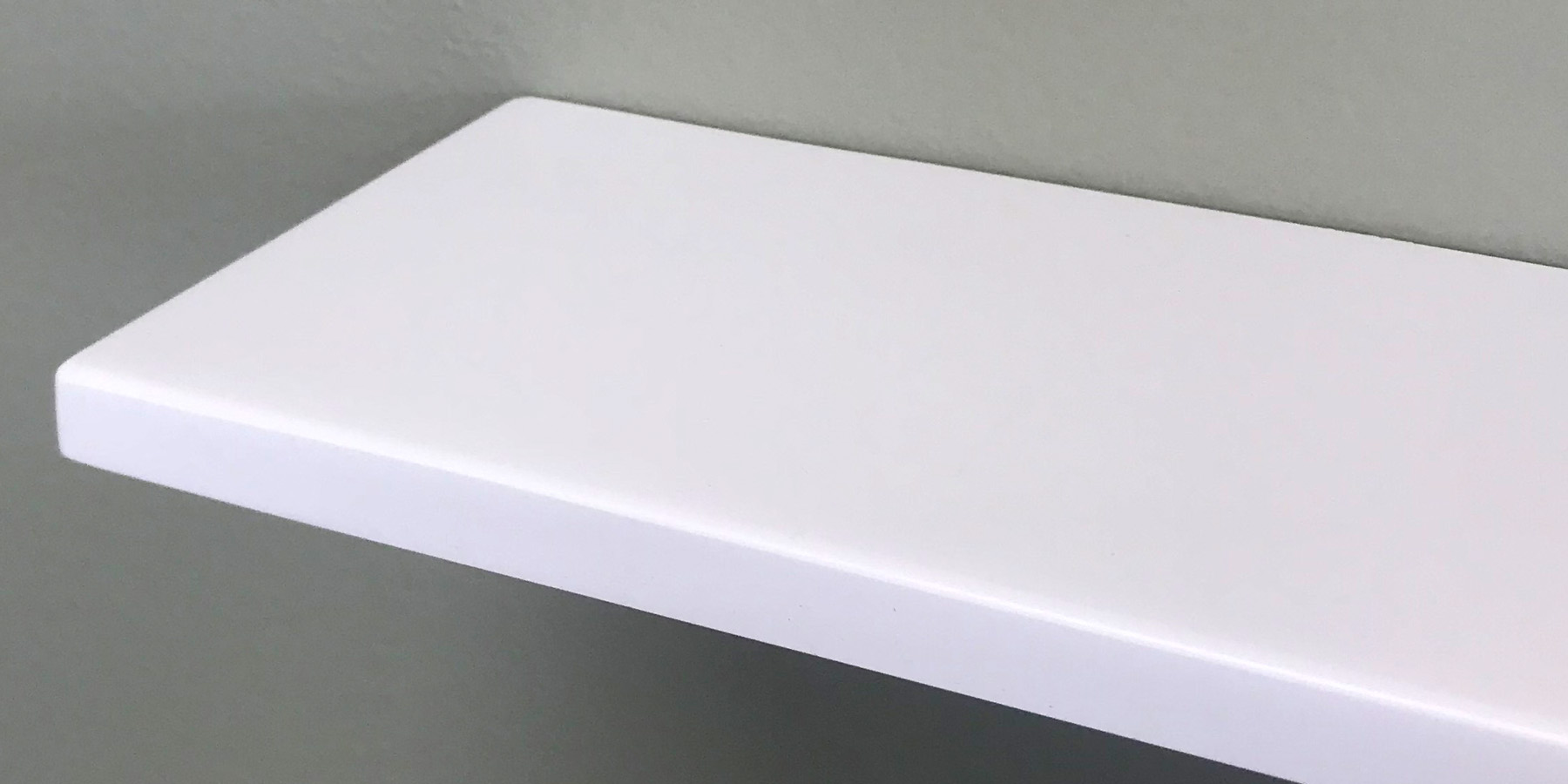The image showcases a sleek, floating white shelf or bench affixed to a textured, medium-gray wall. The wall appears to be painted concrete. The shelf, which might be crafted from either painted wood, hard plastic, or possibly a shiny formica-like material, stretches from the left side of the image but is cut off on the right, leaving its full length indeterminate. Its pristine, glossy surface gives it a modern, minimalist appearance, sitting flush against the wall without any visible means of attachment. The shelf features a subtly curved side and is several inches in width. The clean, sharp lines of the white shelf contrast sharply with the coarse texture of the gray wall behind it, emphasizing its smooth, almost polished finish.